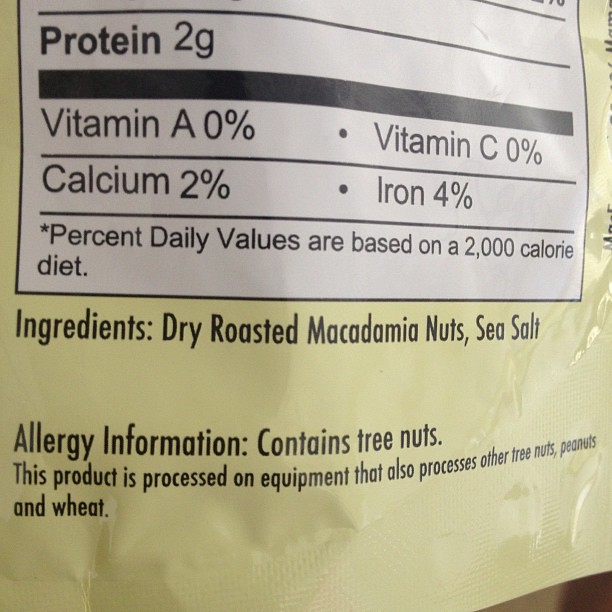The image depicts the lower section of a food package, predominantly yellow with many small creases, likely made of plastic. The lower portion of a white, rectangular nutrition facts label is visible, showing key nutritional information in black text: Protein 2 grams, Vitamin A 0%, Vitamin C 0%, Calcium 2%, and Iron 4%. Beneath this, it states, "Percent daily values are based on a 2,000 calorie diet." Directly below the nutrition label, the black text on the yellow background lists the ingredients: "dry roasted macadamia nuts, sea salt." The packaging also includes an allergy warning, indicating, "Contains tree nuts" and further clarifies, "This product is processed on equipment that also processes other tree nuts, peanuts, and wheat." There's additional, partially visible text on the top right of the image, cut off and not fully legible.